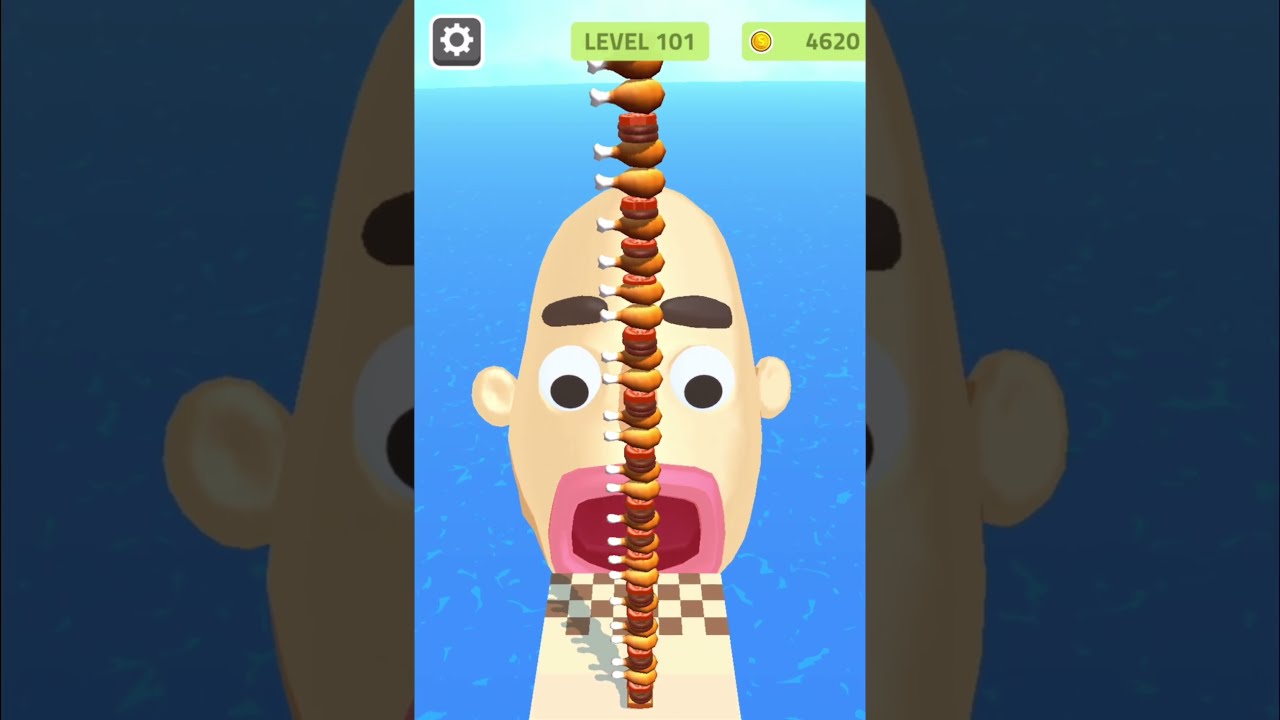The image is a snapshot from a cell phone video game, displaying a vertical rectangular frame centered around a cartoonish, bald man with an exaggeratedly wide, pink mouth and prominent black eyebrows. His mouth is open as if ready to devour the towering stack of chicken wings and hamburgers that rise from the bottom to the top of the frame. In front of him, a black and white checkered pattern, resembling a racing flag or finish line, extends from his mouth, creating a striking focal point. The character stands against a backdrop of a serene blue ocean under a light blue sky, adding a vivid contrast to the scene. 

In the top-left corner, there is a clickable sun or gear icon for settings, and next to it, a green box displaying "Level 101." Beside this, another green box shows a golden coin icon with the number "4620." The sides of the image are grayed out, providing an up-close detail of the central elements. The overall vibrant and engaging layout, coupled with the game's specific markers, indicates this is from an app-based game setup.